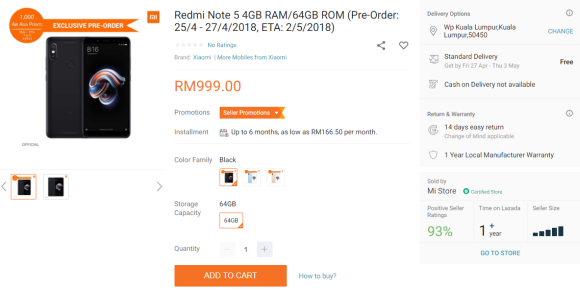This image is a detailed promotional webpage for the "Redmi Note 5" smartphone available for exclusive pre-order. The background of the webpage is white, and the design elements are organized in various colors and sections.

**Top Left Section:**
- An orange ribbon banner with white text that reads "Exclusive Pre-order". This banner extends horizontally from a circular element whose inner details are unclear.

**Top Center Section:**
- To the right of the banner is an orange box containing illegible text.
- The product name "Redmi Note 5" in black, followed by "4GB RAM / 64GB ROM".
- Below, in smaller text: "(Pre-order, 25/04/2018 - 27/04/2018, ETA 02/05/2018)".

**Rating and Brand Information:**
- Below the product information: five gray (unlit) stars with the text "No ratings".
- The text "Brand" with a blurred white word following it.
- A vertical line separating the text "More mobiles from" and a partially blurry word starting with "K".

**Left Section:**
- Below the ribbon, an image of the "Redmi Note 5" showing both front and back views. The phone display's top-left corner shows the time "8:16" and a colorful knotted ball icon.

**Additional Phone Images:**
- Below the main phone image are two smaller images displaying the phone from different angles.

**Pricing and Promotions:**
- On the right, under "Brand", the price is listed as "RM999.00" in orange.
- Below, an "Installments" section with text: "Up to 6 months, as low as RM166.50 per month".
- The "Color Family" section showing three color options for the phone: Black, Blue, and Beige-Yellow.
- The "Storage Capacity" section shows "64GB".

**Cart and Purchase Options:**
- The "Quantity" section, defaulting to "1", with options to adjust quantity.
- An orange "Add to Cart" button.
- A blue "How to Buy" link.

**Delivery Options:**
- "Delivery Options" section includes the address "WP Kuala Lumpur, 50450", with a changeable option.
- Details on standard delivery between Friday, 27 April and Thursday, 3 May, with a "Free" label.

**Return and Warranty:**
- "Return and Warranty" section offering "14 days easy return" and "Change of mind applicable".
- Warranty details: "One-year local manufacturer warranty" shown beside a shield icon.

**Seller Information:**
- "Sold by MI Store" section, featuring a green circle icon indicating "Certified Store".
- Product seller rating: "93%" along with the "One year plus" shop duration.

**Store Navigation:**
- An option to visit the seller store with an increasing-sized box icon and a blue "Go to store" link.

This detailed description encapsulates the comprehensive layout and information of the "Redmi Note 5" pre-order webpage.